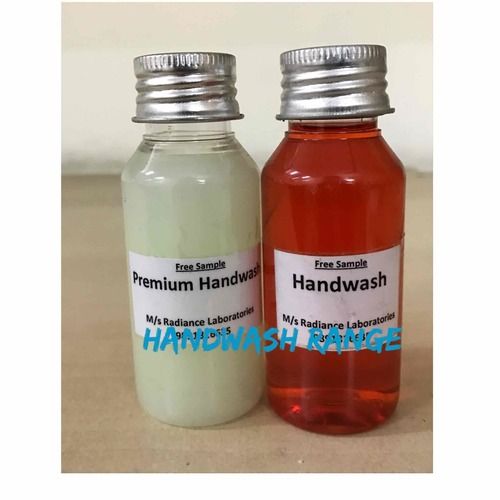This color photograph, taken in portrait orientation with a Photographic Representationalism Realism style, centrally features two small sample bottles of hand wash on a beige wooden surface against a white wall. Both bottles have identical white labels; the left bottle contains a white, milky liquid and reads "Free Sample Premium Hand Wash" in black font, while the right bottle has an orange-red, mostly clear liquid, and reads "Free Sample Hand Wash". At the bottom of the labels, black text reads "M/S Radiance Laboratories" with an illegible number beneath. Superimposed in blue text across the bottom of the labels, it reads "Hand Wash Range". Both bottles are capped with silver aluminum screw-on lids. The image composition accentuates the detailed labeling and the contrasting liquids within the containers.